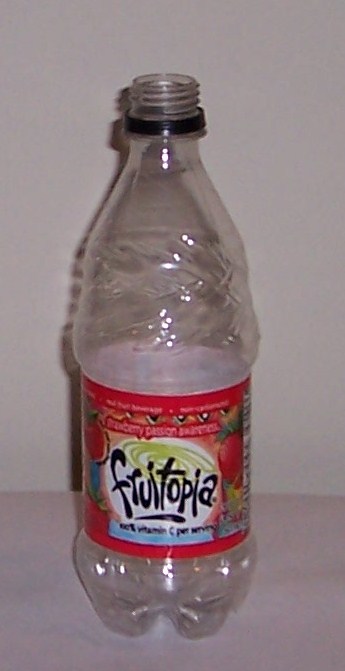This is a close-up image of an empty Fruitopia bottle sitting on a white table, with a plain white wall as the backdrop. The plastic bottle, which holds around 16 to 20 ounces (approximately 250 to 500ml), has a distinctive clear body and a narrow neckline. The design of the bottle includes decorative crosshatches towards the top of the body above the label. The red label, which wraps around the middle without any top label, features the stylized Fruitopia logo in purple letters with green swirls. The label highlights that it provides 100% Vitamin C per serving and is adorned with images of red berries. There is no cap on the bottle, and the shot captures a slight shadow of the bottle against the wall, emphasizing its empty state. The overall composition is simple and minimalistic, placing full focus on the bottle.